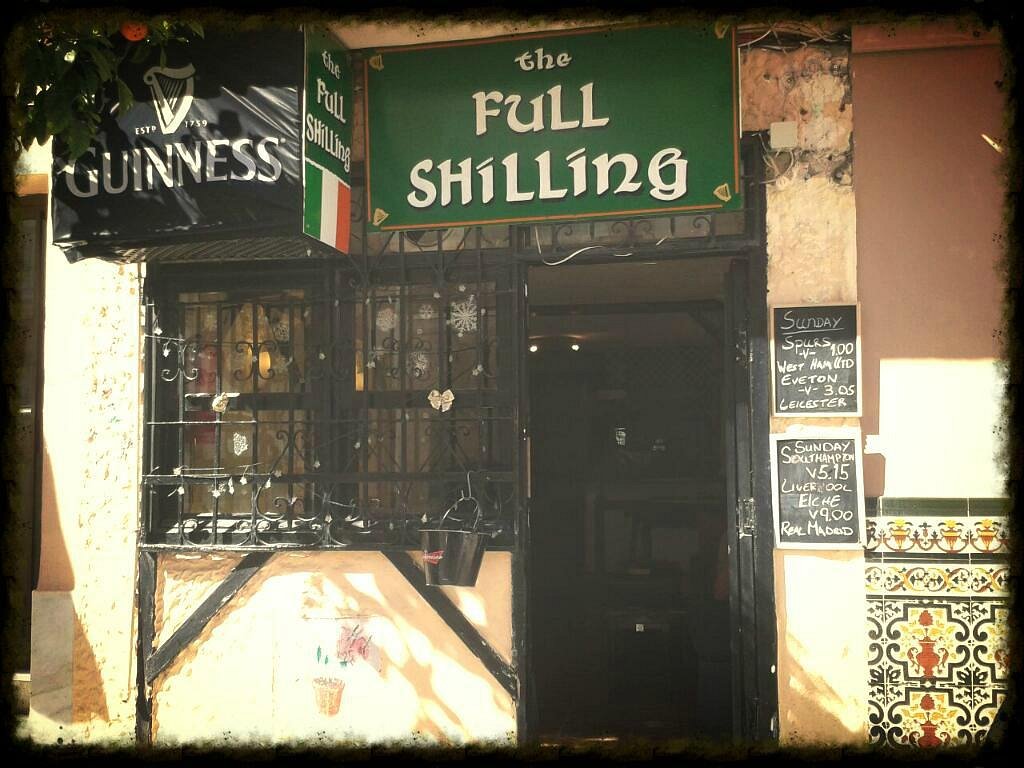The image showcases the exterior of "The Full Shilling," an Irish pub characterized by its rustic charm and welcoming atmosphere. The building features a beige, stone-like facade with contrasting black door frames and metal window coverings, adding to its vintage allure. Prominently displayed is the pub's name in stylish lettering on a green backdrop, flanked by two signs for "The Full Shilling," one above the door trimmed in gold. A black and white Guinness advertisement adds to the authentic pub feel, complemented by a tree with red fruit or flowers nearby.

Black-framed windows and an open doorway reveal a dark interior, suggesting the cozy ambiance within, though details aren't visible due to the bright sunlight outside. On either side of the entrance, chalkboards list upcoming soccer matches, highlighting games such as Southampton vs. Liverpool at 5:15 and Spurs vs. West Ham at 1:00, affirming the pub's role as a hub for sports enthusiasts. Additionally, there's a decorative wall plate featuring a mix of red, black, yellow, and white colors along with various symbols, adding further character to the venue.

The overall setting, including a bucket that might serve as an ashtray, hints at the traditional and social nature of this establishment, likely situated in Ireland, as inferred from its Irish flag and pub-specific details. The adjacent building features a lower tilework of beige, yellow, brown, and black, adding to the quaint, old-world aesthetic of the scene.